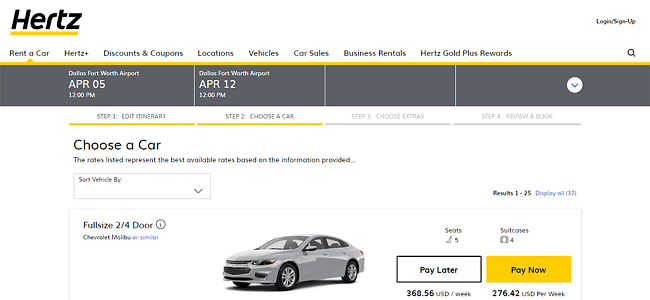Screenshot of a Hertz Rental Car Webpage:

The screenshot captures the Hertz rental car webpage on a clean, white background. In the top left corner, "Hertz" is prominently displayed in bold black letters with a yellow underline. On the far right, options to "Login" or "Sign Up" are visible.

Directly below, a navigation menu is present, with the "Rent A Car" option highlighted. Other menu items include "Hertz," "Discounts and Coupons," "Locations," "Vehicle Car Sales," "Business Rental," and "Hertz Gold Plus Rewards."

Beneath the navigation menu is a dark gray box. On the left side of this box, there are details for a car rental at Dallas Fort Worth Airport, specifying a pick-up date of April 5th at 12 p.m. On the right side, it indicates the return date to be April 12th at 12 p.m. To the far right within the box, there is a white circle with a blue downward arrow.

Below this dark gray box, there’s an option to choose the type of car you wish to rent.